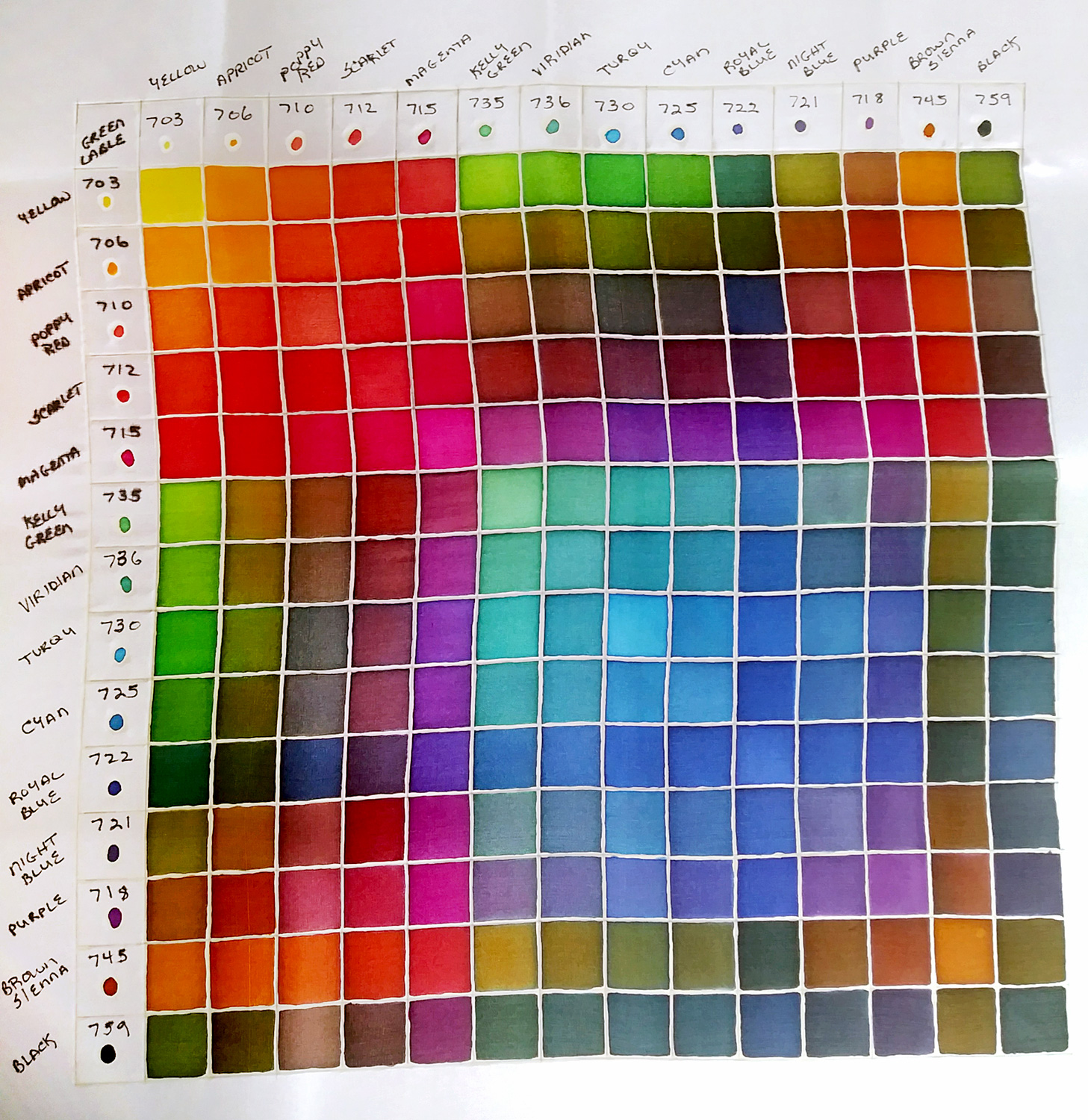This image depicts an intricate, handmade paint mixing chart with a large, detailed grid that resembles a methodical and almost hand-drawn style. Each intersecting box on the grid showcases a unique color created by mixing the colors from the corresponding row and column. Along the top and left edges of the chart, the names and three-digit codes of the base colors are inscribed. For instance, "Yellow 703" appears on both the top and left, indicating the color that appears in the intersecting box within the grid. Each base color is visually represented by a small circle beneath its code both horizontally and vertically. Notable colors listed include "Apricot 706," "Poppy Red 710," "Scarlet 712," "Magenta 715," "Kali Green 735," "Meridian 736," "Turquoise 730," "Cyan 725," "Royal Blue 722," "Night Blue 721," "Purple 718," "Brown Sienna 745," and "Black 759." The fine details of each color blend are methodically organized, demonstrating the nuanced results of combining these watercolors.